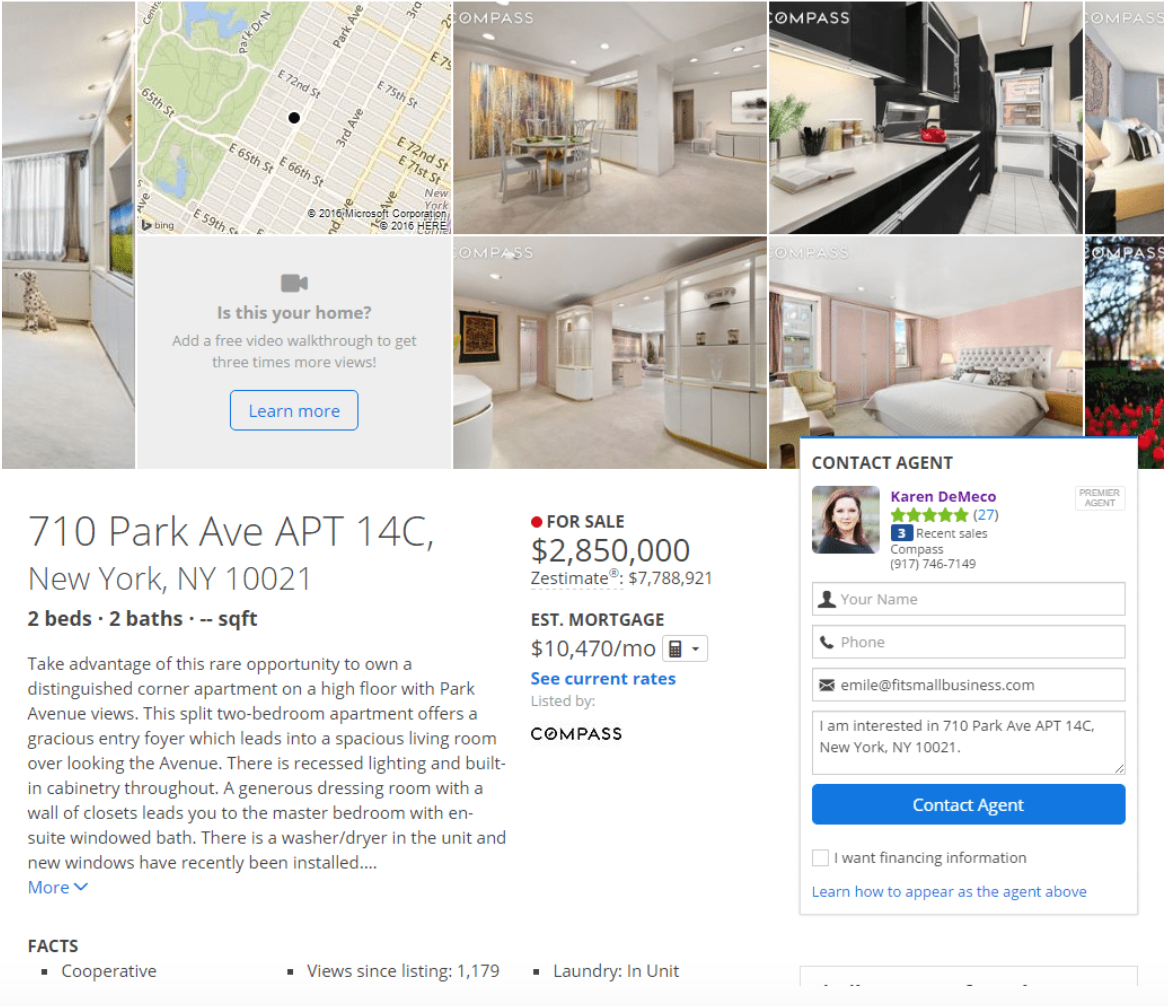This image features a Google Maps still along with several smaller photos showcasing the interior of a luxurious living space. The photos highlight the bathroom, kitchen, and bedroom. The address displayed is 710 Park Avenue, Apartment 14C, New York, New York, 10021. The property is listed as a two-bedroom, two-bathroom apartment with an undisclosed square footage, priced at $2,850,000. Additionally, the image mentions a market value of $7,781,321. A paragraph on the image invites potential buyers to seize the opportunity to own this distinguished corner apartment located on a high floor with views of Park Avenue. The description notes that the apartment features a split two-bedroom layout, a gracious entry foyer, and a spacious living room that overlooks the avenue.